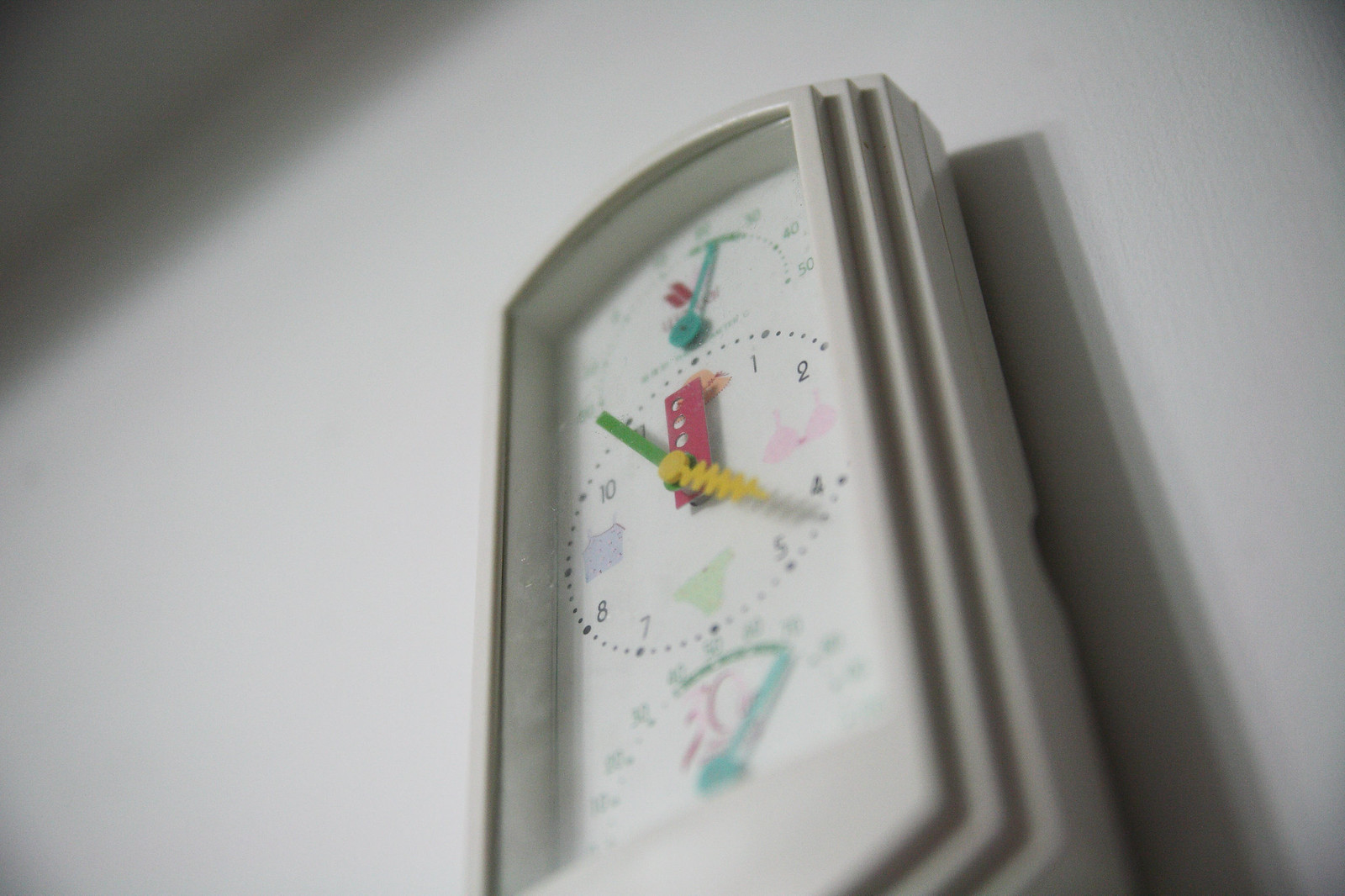The image shows a clock mounted on a gray wall, photographed from a low-angle perspective, giving the impression of looking up at it from the bottom of the wall. The clock is slightly tilted to the left. Its frame appears to be made of gray plastic, while the inner face is white. Unique design elements include a semicircle at the top, a full circle in the center, and another semicircle at the bottom.

The central circle functions as the clock face, with some numbers replaced by various images. The number 12 is obscured, but the numbers 1 and 2 are visible. At the 3 o'clock position, a pink bikini is depicted, followed by the numbers 4 and 5. The 6 o'clock position features an image of a green bikini bottom. Continuing around the clock, the numbers 7 and 8 are present, while the 9 o'clock position shows a blue tank top. The sequence is completed with the numbers 10 and 11. The clock hands are pointing to 4 o'clock.